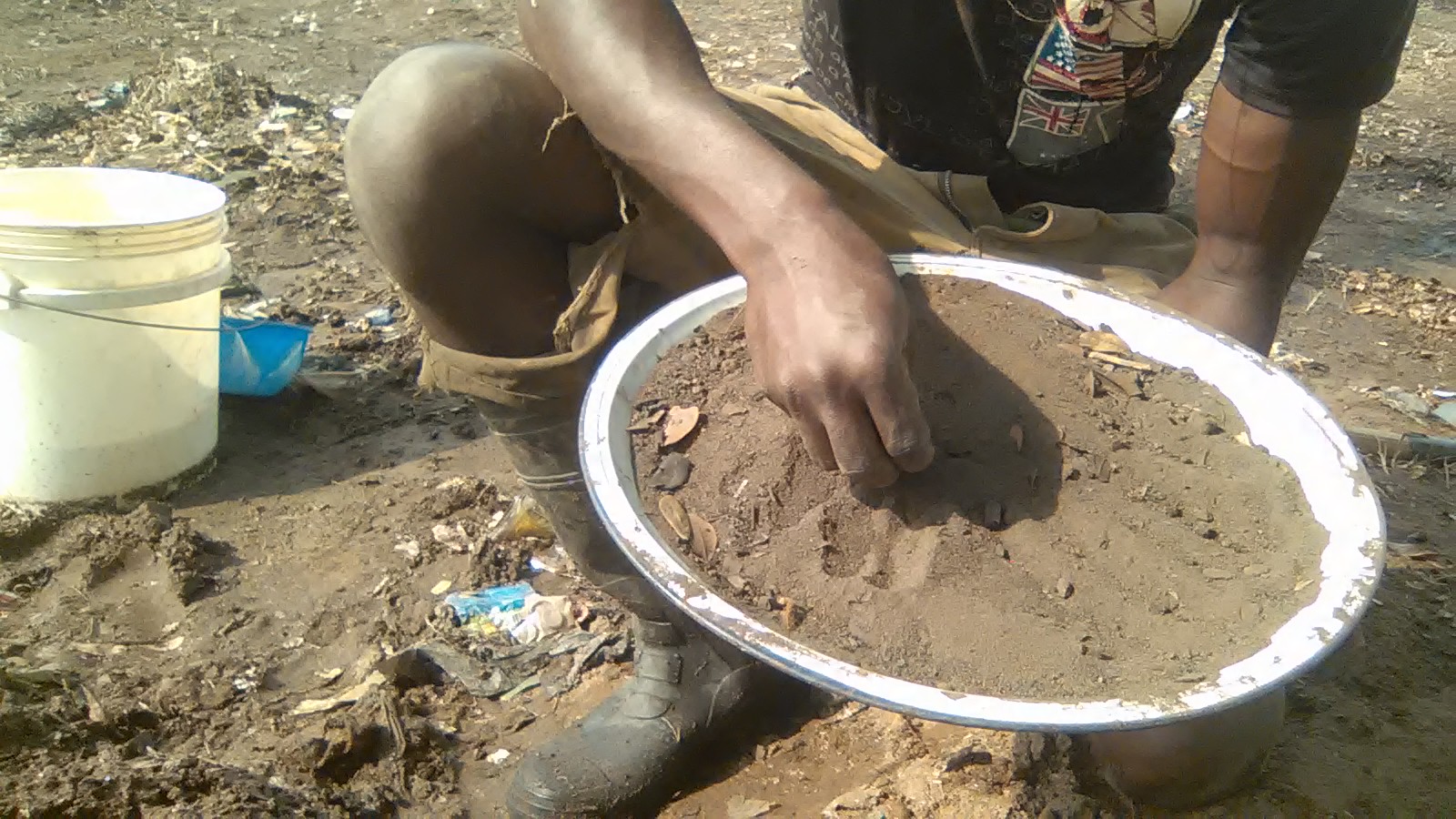A dark-skinned individual is captured in this image, kneeling on the ground and wearing a black t-shirt partially obscured by an intricate design featuring both the American and Australian flags. They sport torn, unzipped pants, with the right knee completely blown out, tucked into rugged rubber boots. Beside them, a white bucket rests on the ground. The person is sifting through fine-grained tan sand with visible debris, using a porcelain-covered pan and their right hand to carefully scrape through the material. The litter in the sand, comprising both biodegradable and man-made items, underscores the pervasive presence of trash in the area.